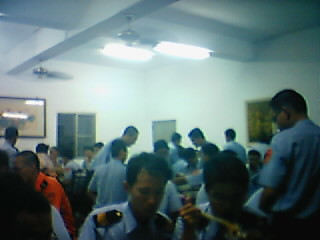This grainy, old photograph, likely from the 70s or 80s, captures a gathering of men in a spacious, brightly lit room. The setting appears to be a police station or an event hall, characterized by high white ceilings with overhead fluorescent lights. The room is decorated with a few pictures and has a couple of windows. 

The men, predominantly in police or military-style uniforms with distinctive shoulder badges, create an impression of being part of an official or formal event. Among the uniformed individuals, a few stand out in orange jumpsuits, possibly indicating roles as workers or crew members in a more hands-on capacity, perhaps from a ship or cargo vessel. The diversity among the men hints that they could be of different nationalities, possibly from Mauritius, Malaysia, or another Asian region. The overall ambiance and structural elements like ceiling beams and struts suggest a utilitarian environment, consistent with either a police station, a ship’s dining hall, or a similar institutional setting.